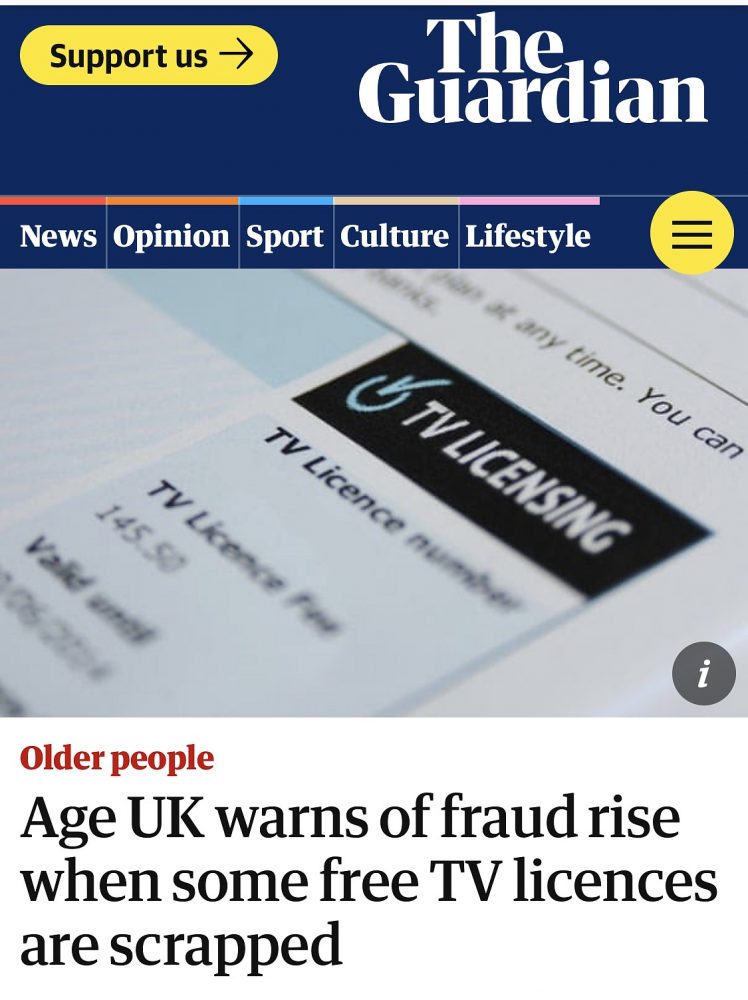Here is a cleaned-up and detailed descriptive caption for the image:

---

The webpage displayed is from The Guardian, characterized by a navy blue background. On the left side of the page, there's a prominent oval-shaped yellow banner with navy blue text that reads "Support us," accompanied by a right-pointing arrow. The Guardian’s logo is centered at the top in large white letters. Below the logo is a colorful horizontal line transitioning from red to orange, blue, beige, pink, and ending with a fine blue line. 

On the left side under this line, navigational links in white text read: "News," "Opinion," "Sport," "Culture," and "Lifestyle." On the right, there is a yellow circle with three horizontal navy blue lines, indicating a menu icon. 

Descending from the primary navy blue section, the background shifts to a shaded gray. There is partial text visible which appears to pertain to TV licensing, displaying a blue semi-circle with a check mark to the left. This section reads partially due to being cut off, but includes mentions of "TV licensing," "TV license number," and "145.50.", with a small gray circle containing a white "i."

Below this gray section, the background turns white with the heading "Older People" in red. Underneath, in larger black text, the article title reads: "Age UK Warns of Fraud Rise When Some Free TV Licenses Are Scrapped." This segment appears to be the focal point of the article.